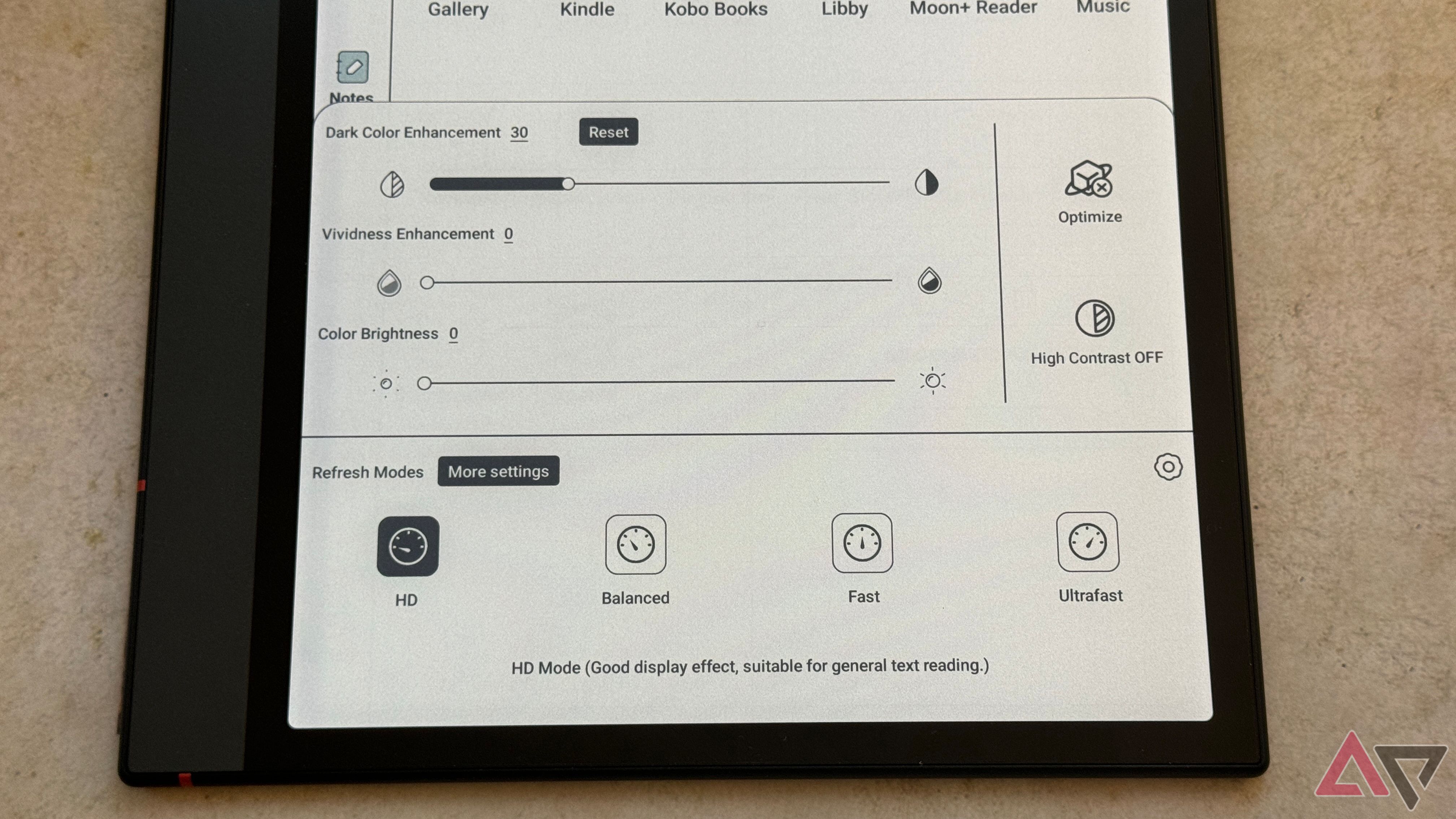In this image, a tablet rests on an undetermined surface displaying a comprehensive settings menu. The screen is busy with textual information and various interactive elements.

At the top, a header showcases a list of applications: "Gallery," "Kindle," "Kobo Books," "Libby," "Moon Plus Reader," and "Music." Below these, another section is titled "Notes."

The screen is divided into multiple sections featuring adjustable settings. The first section includes "Dark Color Enhancement 30" with a horizontal adjustment bar and an option to "Reset." Next, there's "Optimize," followed by "Vividness Enhancement 0" paired with another horizontal bar for adjustments.

Proceeding down the screen, there is a section labeled "Color Brightness 0," again paired with a horizontal adjustment bar.

On the far right side, under "High Contrast Off," the menu offers options for "Refresh Modes," "More Settings," and "HD in Blackprint." The refresh modes are categorized as "Balanced," with an icon of a clock displaying 12 o'clock labeled "Fast," and another clock showing a time close to 1 o'clock labeled "Ultra Fast."

Below these options, a descriptor reads, "HD Mode, Good Display Effect, Suitable for General Text Reading." Additionally, a gear icon, likely indicating more settings, is positioned on the far right side of the screen.

The tablet itself features a black border, while the background of the displayed menu is either white or a light gray, creating a stark contrast with the black text.